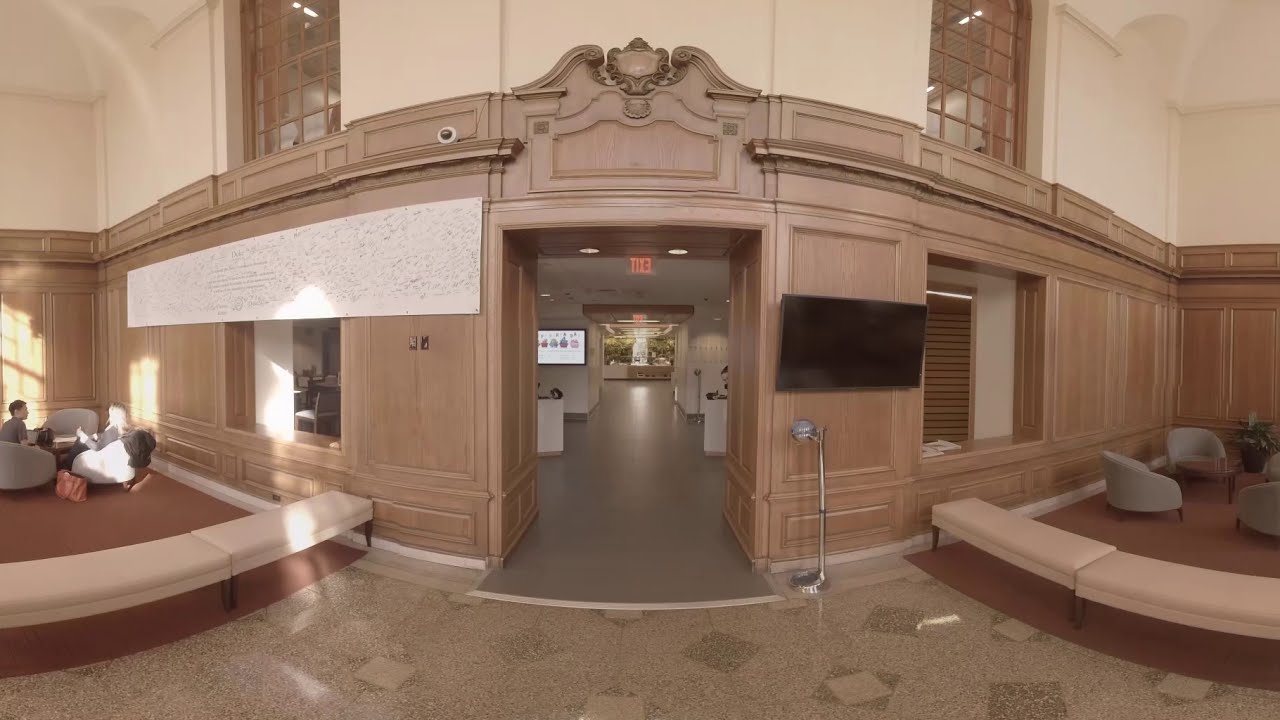The photograph depicts the interior of a modern, two-story lobby or waiting area, potentially in a hotel, courthouse, or hospital. The space is characterized by light brown wood paneling and cream-colored upper walls. Centrally positioned is an entranceway flanked by windows and lower ledges, while above the doorway hangs a prominent red "EXIT" sign. On the right side of the image, a black, unlit TV screen is mounted on the wall. The lobby features various seating options, including gray chairs and cream-colored benches, with people occupying some of the chairs. The floor is a mix of tan, beige, and brown colors, adding warmth to the setting. Additionally, towards the background, there seems to be another TV screen and white display stands, possibly indicating an area for brochures or informational material. Overall, the area stands out for its spacious, modern design, with natural wood accents and practical furnishings, providing a welcoming atmosphere.